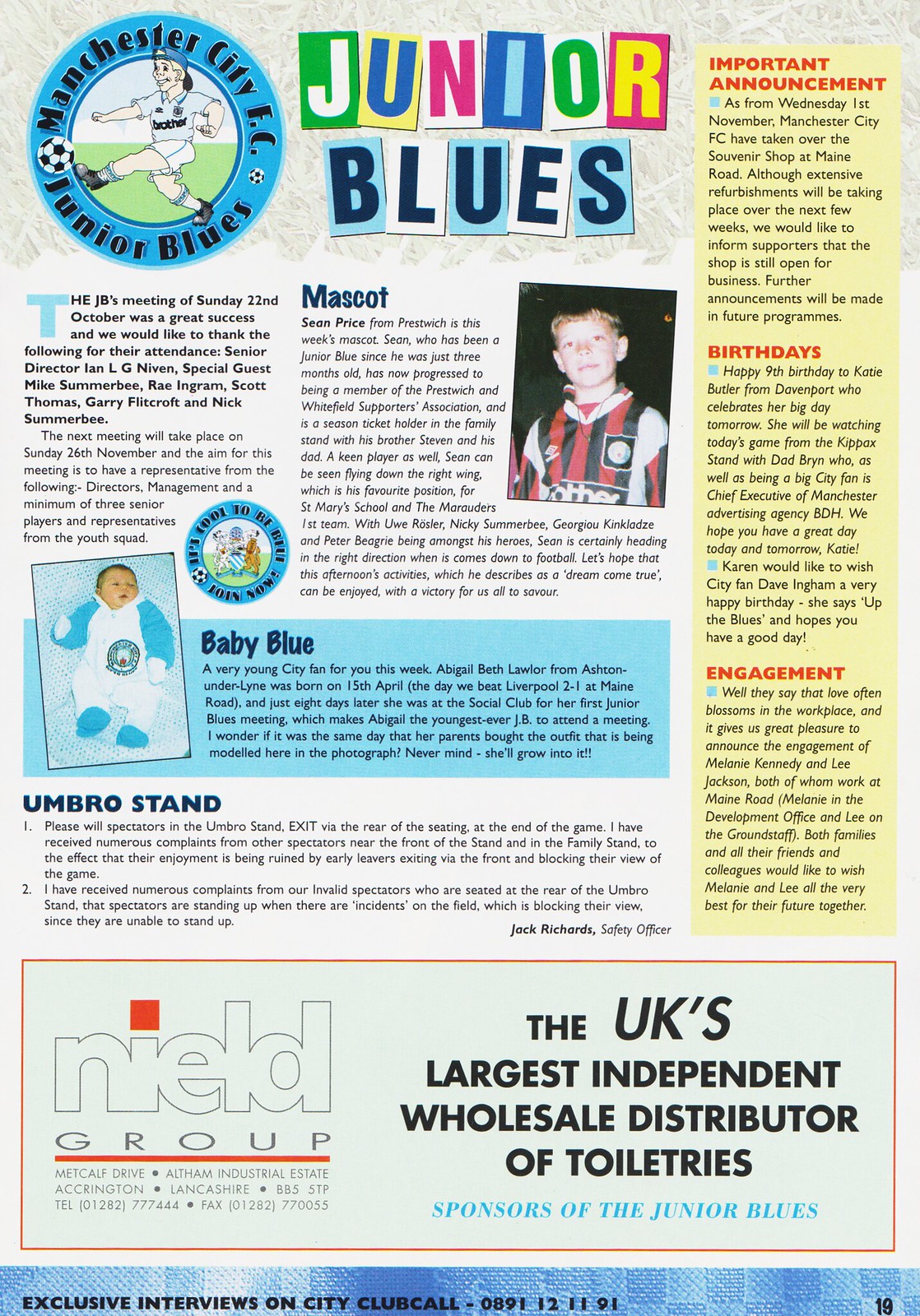The image features page 19 of the 'Junior Blues' magazine, topped with the text "Junior Blues" spelled out in colorful, lettered rectangles. A round logo in the top left corner reads "Manchester City FC Junior Blues" and includes an illustration of a boy in a light blue shirt, white shorts, and a backwards blue cap kicking a soccer ball, with "brother" printed on his shirt. The page highlights several sections: a photo of mascot Sean Price from Prestwich, labeled "mascot," and a baby named Abigail Beth Lawler from Ashton-under-Lyne born on April 15, tagged "baby blue." Additionally, there is a yellow panel on the right side for important announcements, birthdays, and engagements. At the bottom, an advertisement for the Nield Group, identified as the UK's largest independent wholesale distributor of toiletries, includes contact details and boasts of their sponsorship of the Junior Blues.